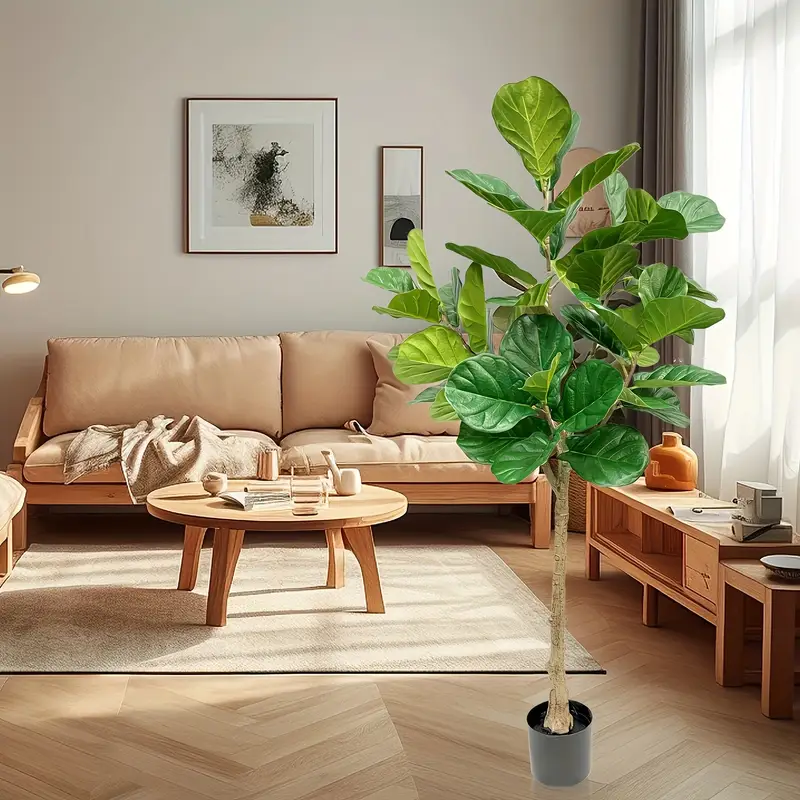The image captures a modern living room with a Scandinavian design. The room features neutral-toned parquet flooring and a tan beige couch, complemented by matching beige cushions. A prominent tree-like plant with broad green leaves, housed in a small gray pot, stands in the foreground, appearing somewhat out of scale. A circular wooden side table with four legs sits atop a beige rug in the center of the room, adorned with an orange vase and decorative boxes. The room is bathed in natural light streaming through white curtains on the right, which highlights a shelf holding various artifacts. Two abstract paintings hang on the wall, one square and one rectangular, both incorporating black elements but maintaining a subdued palette. A table lamp to the left casts a warm white glow, enhancing the room’s inviting atmosphere. The overall scene is characterized by its minimalist decor and neutral colors, with the vibrant green plant serving as the focal point.